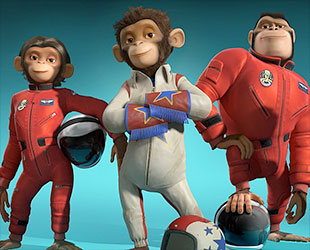In a vibrant, blue-to-deeper-ocean-blue gradient background, three animated monkeys stand in human-like poses, clad in sport or stunt-type suits. The left monkey, possibly female, wears a red suit extending down to her wrists and ankles, holding a helmet under her left arm. The central monkey, exuding a sense of attitude, dons a white suit accented with red and blue stars around the wrists. His arms are crossed over his chest, and his head tilts slightly to the left as he gazes ahead. The rightmost monkey, the largest, is also in a red suit similar to the left monkey but subtly orangish, with a distinguishing blue badge featuring white wing-like designs. This monkey stands confidently with one knee up, foot on a helmet, and his right hand resting on his raised knee, looking out with his chin elevated. Each suit leaves their hands and feet uncovered, emphasizing their readiness for a sporting challenge or a daring stunt.